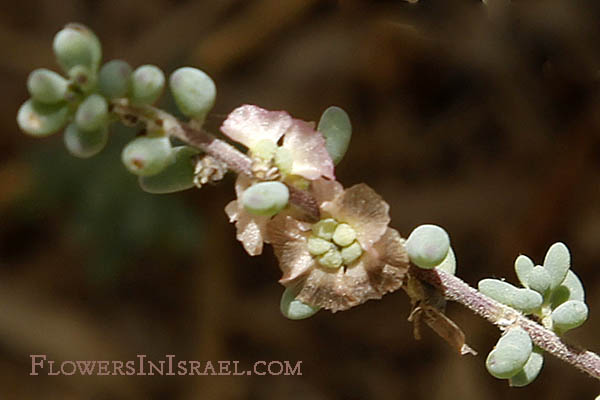In this watermarked photograph, labeled flowersinisrael.com in the bottom left corner, the focal point is a striking plant branch that stretches from the lower right to the top left of the frame. The branch itself is light brown, and it is adorned with succulent-looking, bean-shaped green nodules—about eight in total—that are nestled on either side of the branch. Some of these nodules have unfurled into delicate, cream-pink flowers with clusters at their centers, resembling small, dull purple blooms. The background is a dark, blurred mix of browns, black, and hints of orange and cream, providing a soft contrast that makes the branch and its vibrant details stand out prominently. The overall setting suggests a hardy plant species, fitting for the arid environments typical of Israel.